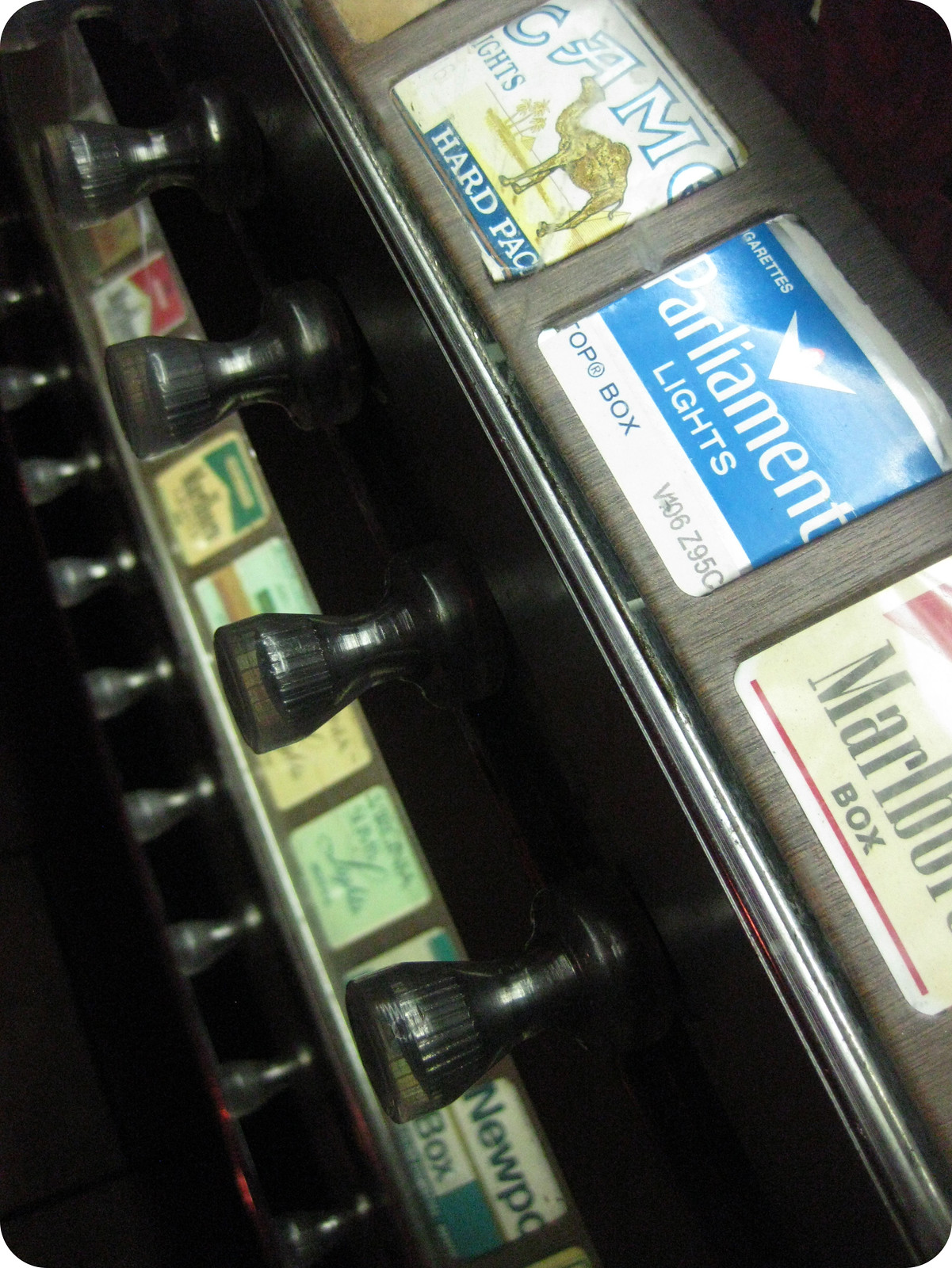This close-up image features an old-fashioned cigarette vending machine, evocative of bygone eras. The machine prominently displays several packs through various windows, including a Camel Lights hard pack in the upper right, a Parliament Lights box in the middle right, and a Marlboro box towards the bottom right. Below these windows is a row of blurry and obscured cigarette packs, with identifiable brands such as Newports amid other choices. The machine is equipped with semi-transparent knobs, likely operated to dispense the desired pack, reminiscent of a bygone era. The nostalgic appearance and design of the machine, strikingly similar to a jukebox, adds a poignant touch of history, reminding us of a time when such machines were commonplace despite the inherent risks they posed.